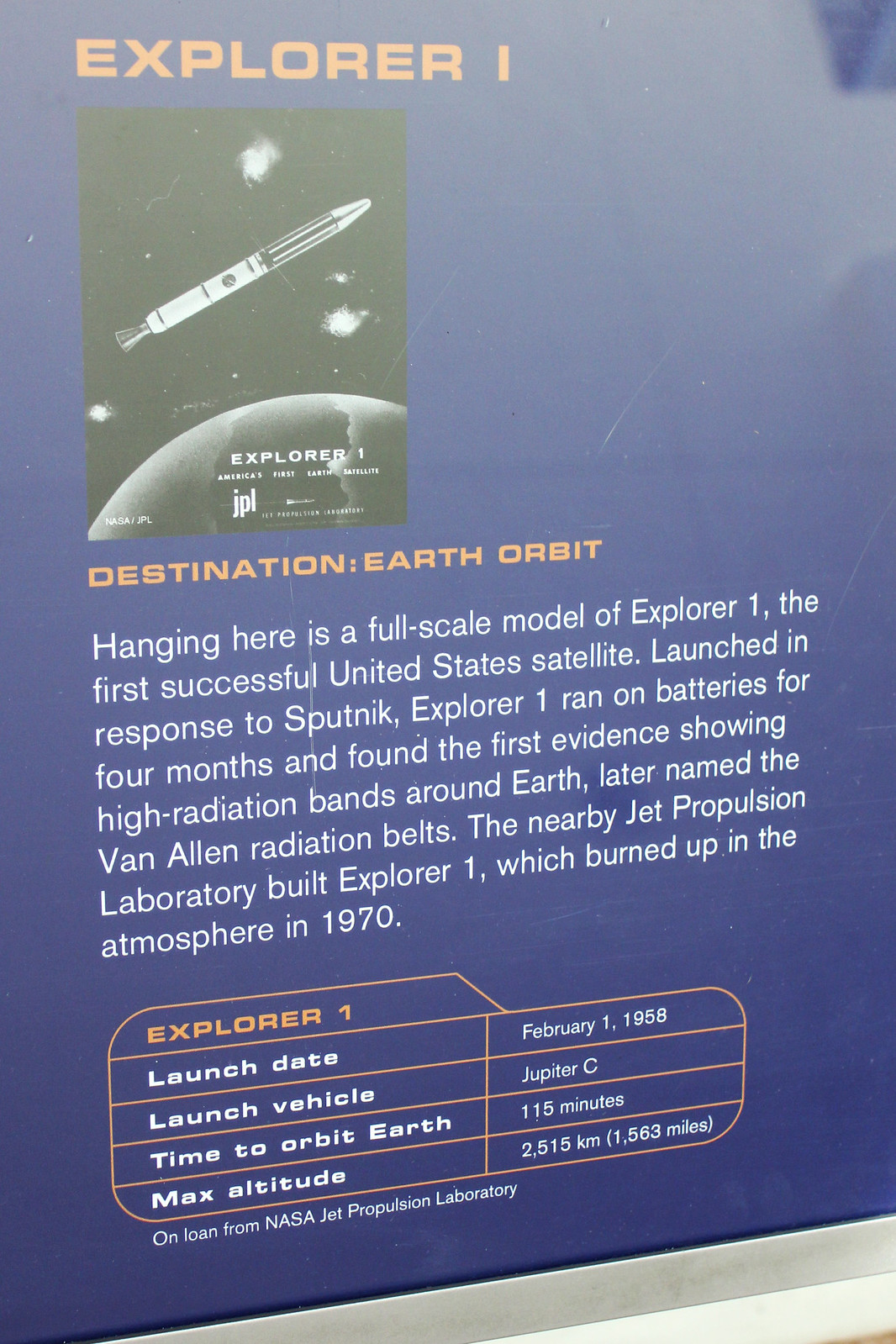This exhibit sign, displayed most likely in a space museum, provides detailed information about Explorer 1. Predominantly blue with white and orange lettering, the sign features a black-and-white image of the rocket. It prominently states "Explorer 1," accompanied by the phrase "Destination: Earth Orbit" in orange font. The sign explains that hanging here is a full-scale model of Explorer 1, the first successful United States satellite, launched in response to Sputnik.

Explorer 1, which resembles a small rocket, ran on batteries for four months and discovered the high radiation bands around Earth known as the Van Allen radiation belts. Built by the nearby Jet Propulsion Laboratory, Explorer 1 ultimately burned up in the atmosphere in 1970. The information panel also details key facts about the satellite: its launch date was February 1, 1958, it was launched using a Jupiter-C vehicle, it took 115 minutes to orbit Earth, and it reached a maximum altitude of 2,515 kilometers or 1,583 miles.